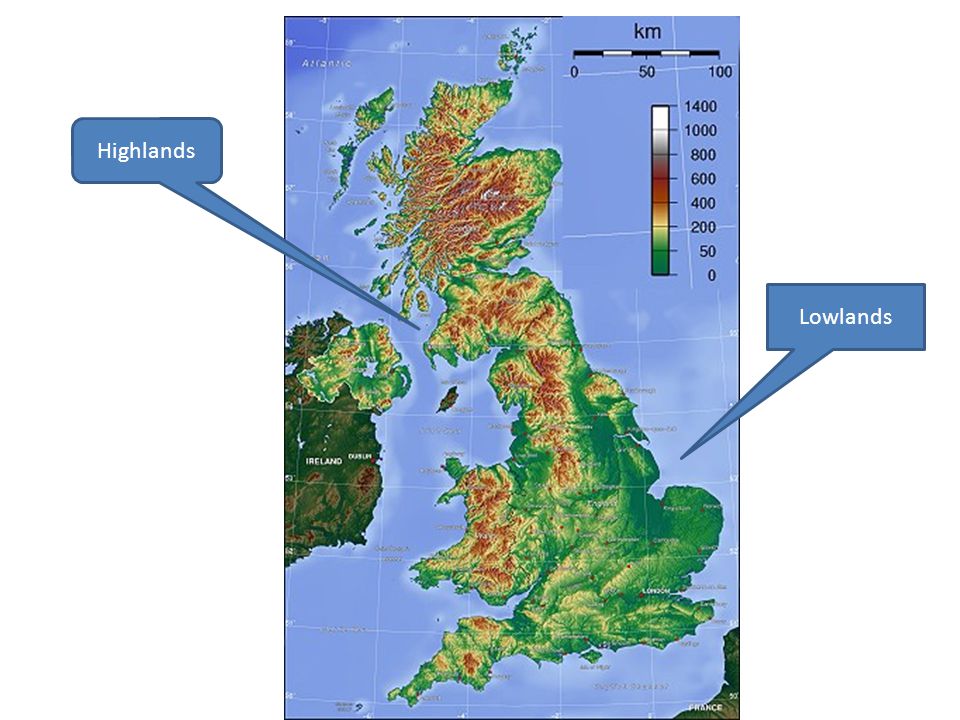This is a detailed physical map of an elongated island, primarily covered with color-coded areas in green, red, and yellow. The landmass is surrounded by the blue of the ocean, which represents water. To the left of the main island, there is an adjacent land formation, half-visible in the image, likely representing Ireland. Two areas within the island are explicitly marked: a blue pointer on the left identifies the "Highlands," while another blue pointer on the right identifies the "Lowlands."

Towards the upper right corner of the map, there is a black and white distance scale marked with '0', '50', and '100' and labeled 'KM.' Below this horizontal scale, there is a vertical elevation legend with various color shades, starting from white at the top, followed by red, yellow, and green. The elevation markings read from top to bottom: '1400', '1000', '800', '600', '400', '200', '50', and '0'. The map is taller than it is wide, creating a vertical orientation that emphasizes the height differences in the terrain.